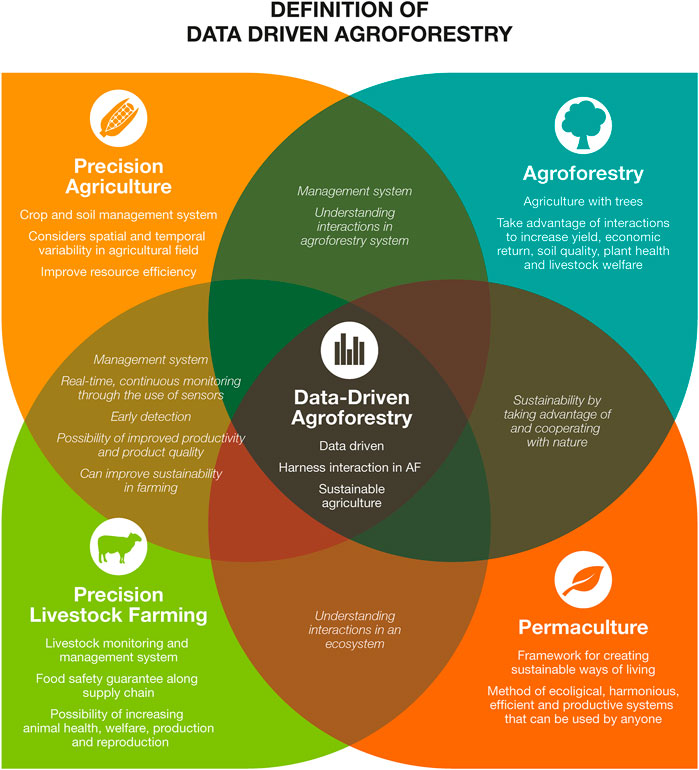This image is a detailed Venn diagram chart titled "Definition of Data-Driven Agroforestry." The chart showcases four transparent, overlapping leaf-like shapes, each pointing towards one of the four corners of a white background square. 

- The **upper left leaf** is bright orange featuring an ear of corn inside a white circle. Below this, it reads "Precision Agriculture" in bold white lettering, followed by four lines of smaller white text.
- The **upper right leaf** is blue, displaying a leafy tree inside a white circle. Beneath it, the title "Agroforestry" is written in bold white letters, followed by a subheading and a paragraph of small white text.
- The **lower left leaf** is bright lime green with a cow icon in a white circle. Below this is "Precision Livestock Farming" in bold white lettering, with three paragraphs of smaller white text.
- The **lower right leaf** is dark orange, showcasing a leaf on a stem inside a white circle. Underneath, "Permaculture" is boldly written in white, accompanied by two paragraphs of small white text.

Where these colorful leaves overlap, the colors darken, interlocking towards the center. In the central area, the overlapping leaves form a darker multi-colored oval. Here, a white circle contains a symbol representing data-driven processes (five vertical lines), encircled by bold white text that states "Data-Driven Agroforestry." Below this, three lines of smaller white text, specifying "Data-Driven, Harness Interaction to AF, Sustainable Agriculture," are present.

Each leaf section contains text specific to its category, contributing to the comprehensive depiction of data-driven methodologies in different agroforestry fields.